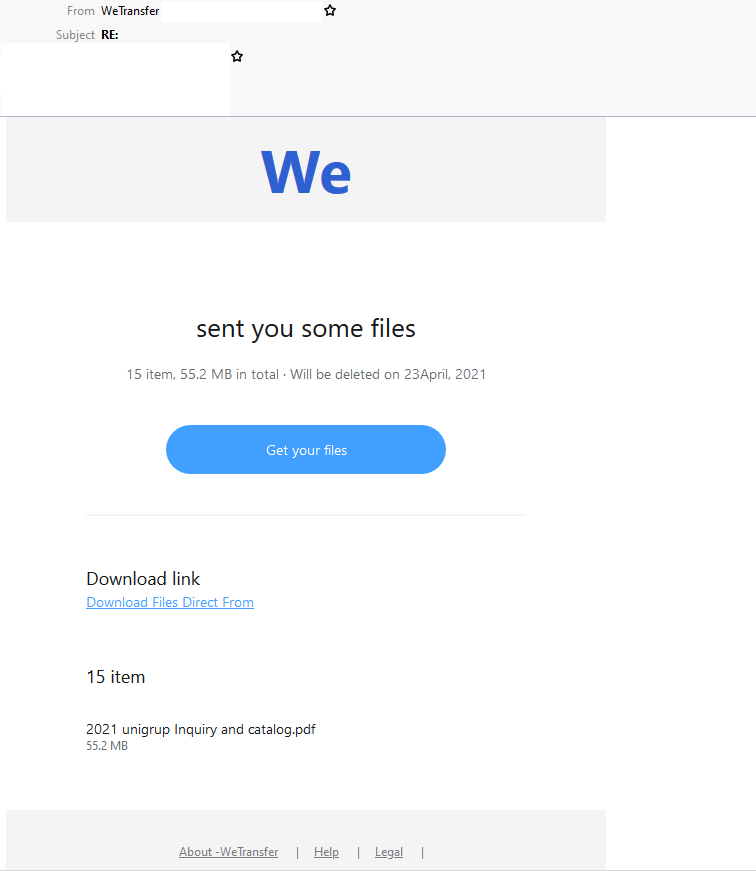### Captured Image Description:

The image features a website interface with several distinct sections.

1. **Header:**
   - **Background:** Light gray, serving as an overlay against the initial website.
   - **Text:** 
      - Left side: "from" in regular gray.
      - Right side: “WeTransfer” with specific styling: Capital 'W,' lowercase 'e,' capital 'T,' lowercase 'ransfer' in darker gray.

2. **Obscured Personal Information:**
   - **White Rectangular Area:** Blurring out personal information in a large rectangular region.
   - **Star Icon:** Black outline star towards the right of this area.
   
3. **Subject Area:**
   - **Text:**
      - Left side: "subject" in gray.
      - Right side: “RE:” in bold, black, capital letters.
   - **Additional Obscured Information:** Another larger white rectangular area blurring out more personal information.
   - **Star Icon:** Black outline star towards the right again.

4. **Main Content:**
   - **Banner:** 
      - **Background:** Medium gray (darker than the header).
      - **Text:** "We" with a capital 'W' in blue, bold lettering, centered.
   
   - **Message Area:** 
      - **Background:** White.
      - **Main Message:** In black font, "sent you some files."
      - **File Details:** In small gray font, "15 items, 55.2 MB in total • will be deleted on 23 April, 2021."
   
   - **Download Button:**
      - **Shape:** Oval.
      - **Background:** Blue.
      - **Text:** In white, "Get your files," centered.
   
   - **Divider Line:** Gray line serving as a divider below the download button.
   
   - **Download Link:**
      - **Text:** 
         - Left side: "Download link" in black.
         - Below it: A clickable URL styled as underlined blue text, "download files direct form."

This detailed description captures the visual elements and text displayed in the image of the website, emphasizing the structure and key components of the layout.